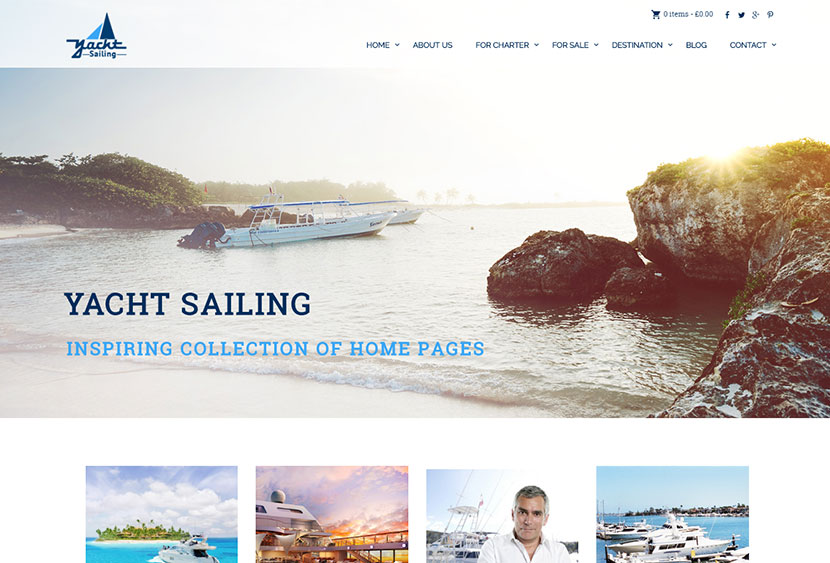Homepage of "Yacht Sailing" Website

In the top left corner, the website's logo, "Yacht Sailing," is prominently displayed in a dark blue font, complemented by a stylized yacht sail in light and navy blue. The main feature image showcases two large, white yachts accented with blue highlights, docked near the shoreline. The scene includes a sandy beach, gentle waves, and bright sunlight. In the background, one can notice rocks and distant islands.

Below the main image, a caption reads "Yacht Sailing, inspiring collection of homepages." Additionally, there are four smaller images at the bottom. These images include: 

1. A powered sailing boat heading towards an island.
2. A mid-sized cruise ship.
3. A man in a polo shirt standing on his yacht.
4. Four yachts docked at a harbor.

All images are taken during daylight.

At the top of the page, a navigation menu features categories such as Home, About Us, For Charter, For Sale, Destination, Blog, and Contact, each with a dropdown arrow indicating additional options. On the right side of the navigation bar, there is a cart icon displaying "Zero Items" and a monetary value of "60" (currency unspecified). Social media icons for Facebook, Twitter, and Gmail are also available for easy contact.